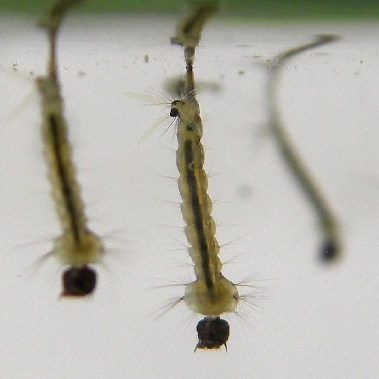The image depicts a close-up view of three tan-colored caterpillars, each adorned with hair-like tentacles along their bodies and a black stripe running vertically from head to tail. The caterpillars appear to be hanging against a white background. The central caterpillar is in sharp focus, showing a distinct rounded, dark head and a narrow tail. To the left of the main caterpillar is a slightly smaller and more blurry caterpillar that seems to mirror the central one, suggesting it might be a reflection. To the right, there's a third caterpillar, also slightly curved and more out of focus, visible primarily as a shadowy shape. The overall composition gives an impression of a detailed, microscopic view where the minuscule details and textures of the caterpillars are emphasized, especially the translucent bodies and the dark line running through their middles.